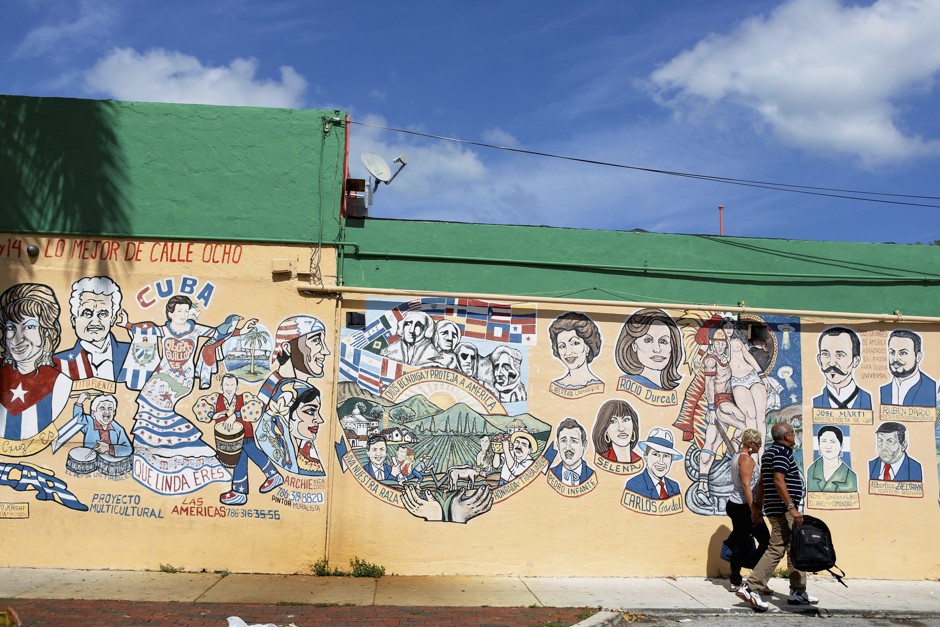This image showcases a vibrant mural painted on the side of a building. The building's wall, on which the mural is painted, is white while the top section above the mural is painted green. The mural itself is a rich tapestry of cultural pride, featuring various faces and symbols representing Cuban and Hispanic American heritage.

On the left side of the mural, the word "Cuba" is prominently displayed along with the phrase "Protecco Multicultural Las Americas." Below, several faces are depicted, representing the diverse cultural background of the community. On the right side, more faces are featured, each labeled with names of significant Hispanic figures. Included among these are the famous singer Selena, the legendary tango performer Carlos Gardel, and a woman labeled Rocío Dúrcal.

Additionally, the mural incorporates a seal that includes images of fields and a version of Mount Rushmore. However, instead of the U.S. presidents, this version showcases renowned Hispanic personalities, further emphasizing the celebration of Hispanic cultural contributions. The overall composition and detailed depictions serve as a striking homage to multiculturalism and heritage.